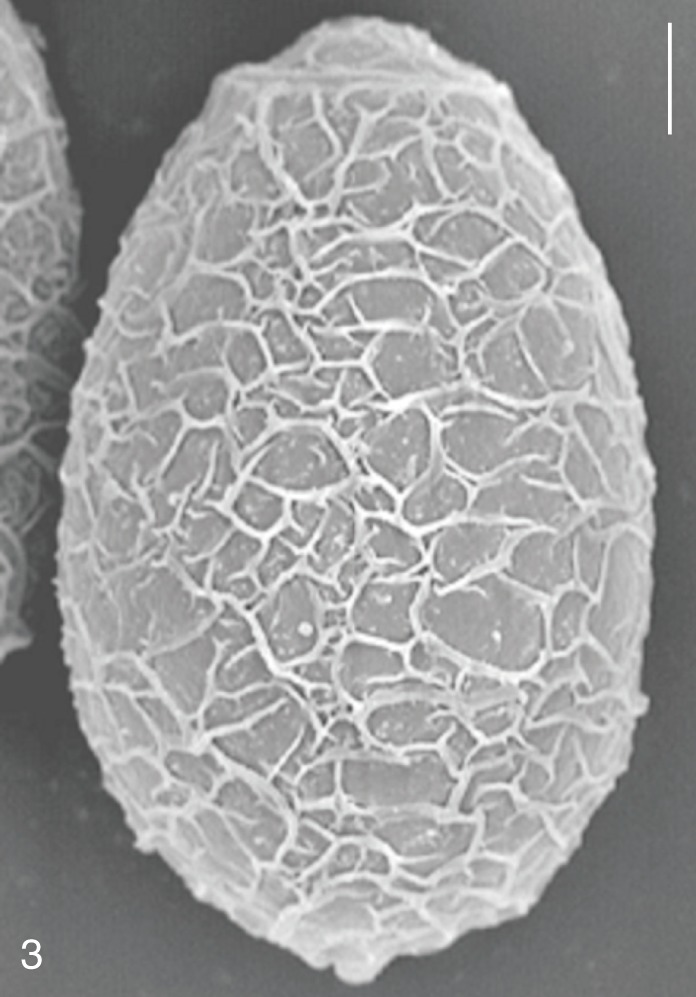This black-and-white photograph, likely taken through an electron microscope, showcases a heavily magnified, egg-shaped object with a complex surface texture. The main subject is an oval, possibly a seed, displayed in a dark gray background. The object is predominantly gray, crisscrossed with intricate, tangled white veins that zigzag across its bumpy surface. The oval shape is not smooth, featuring irregularities where the veins intersect and protrude. In the upper right-hand corner, a distinct white line descends, adding to the intricate detail. The bottom left-hand corner of the image prominently features the number 3. The photograph is taller than it is wide, with no additional text, people, or animals present. Another similar, smaller object is partially visible in the top left-hand corner, sharing the same color and veining pattern.